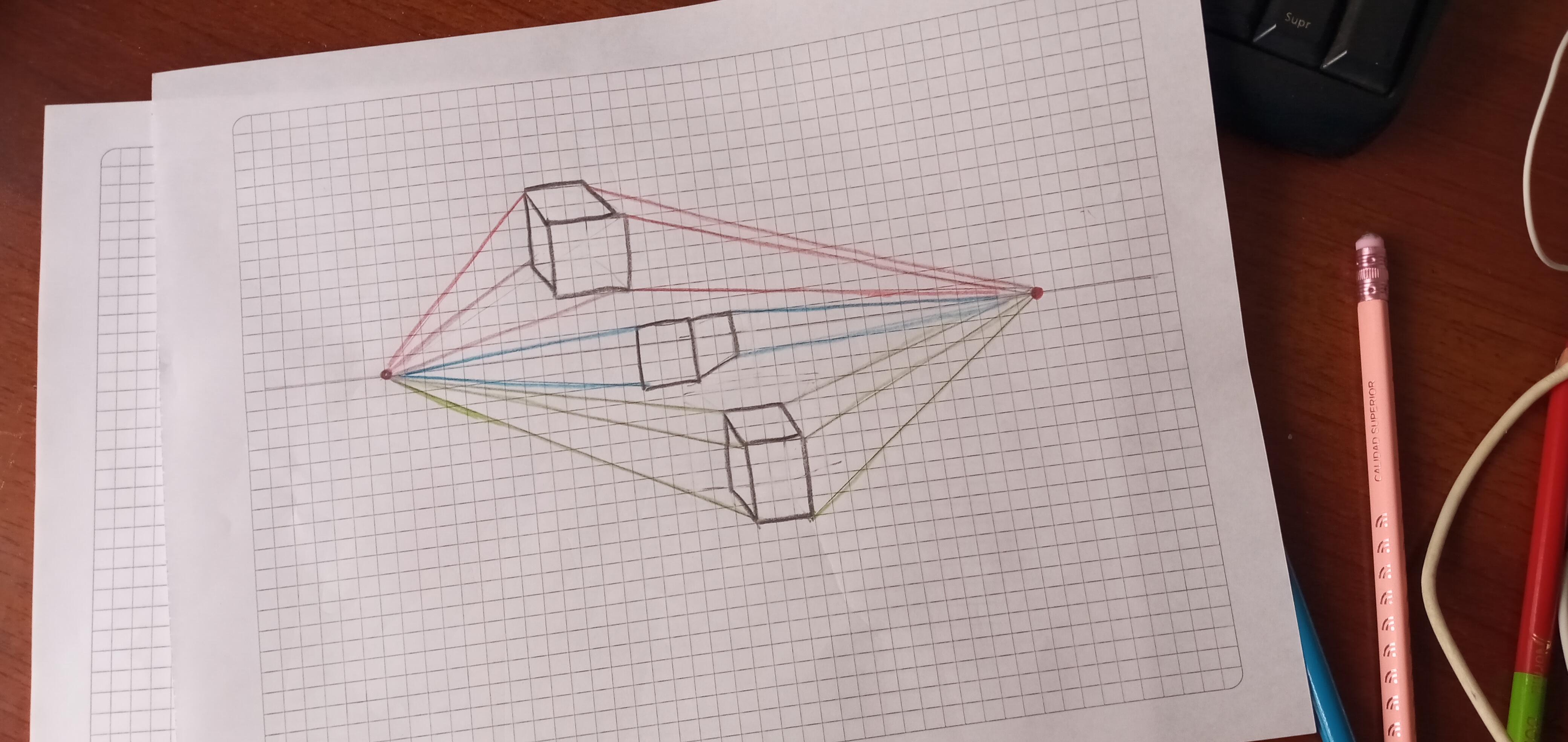On a medium brown wooden desk, two pieces of grid paper are placed neatly. The bottom sheet is almost completely covered, leaving no visible details, while the top sheet prominently displays a meticulously drawn geometric design created with colored pencils. The design features three cubes arranged diagonally from the top left to the bottom right. Each cube is uniquely colored; the top cube is red, the middle cube is blue, and the bottom cube is green. From every point of the cubes, six colored lines extend, converging towards dots positioned on either side of the paper. This elaborate pattern suggests a geometric art piece, possibly intended for use in a mathematical context such as a textbook.

Surrounding the grid papers, various items add to the scene's character. A pink pencil with a matching pink eraser adorned with a repeating design lies nearby. A red marker with a green lid and some white cords, likely belonging to Apple devices, are also present, complementing the organized yet creative workspace.